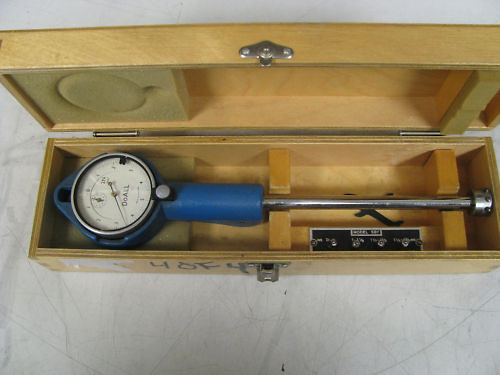The image features a detailed view of a pressure gauge, meticulously enclosed in a custom light brown wooden box with its lid open, revealing the contents. The gauge itself is prominently positioned and appears to be designed for measuring air pressure. Its construction includes a sturdy silver metal base that securely fits into two dedicated wooden slots within the box, indicating that the box was specifically crafted to house this gauge.

A distinctive blue handle, likely made from plastic or rubber, extends from the metal base and surrounds the gauge's face, providing a stark contrast to the white background of the face. The face of the gauge is clearly marked with numbers, lines, and some text, allowing precise readings. A single black hand is present, intended to indicate the measured pressure.

The wooden box is equipped with a silver-colored metal latch, ensuring it can be securely closed when necessary. The entire setup rests on a solid white floor, and the photograph captures the gauge from a top-down perspective, providing a clear and comprehensive view of all its components and their arrangement within the box.